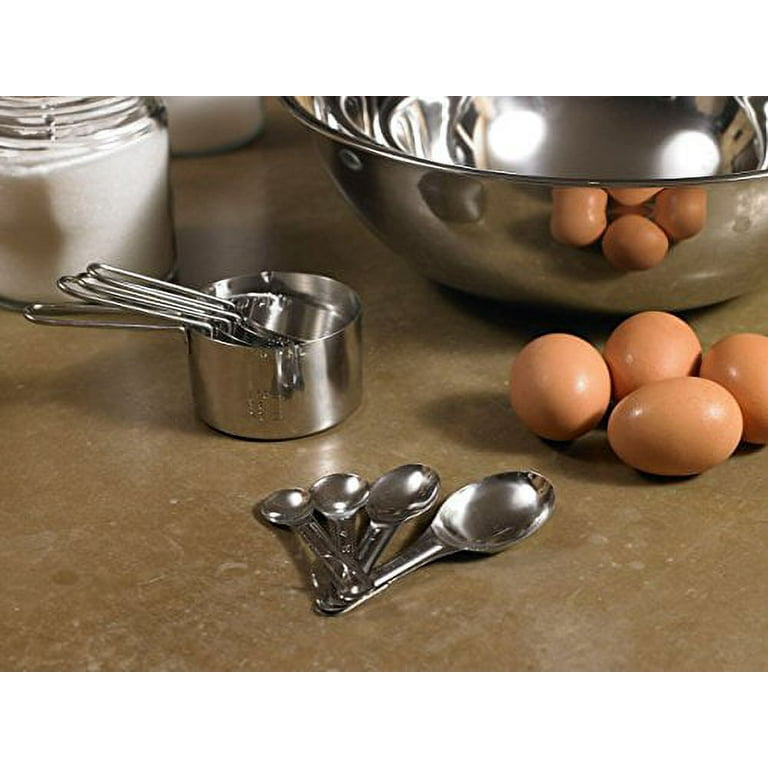The image is a color photograph, likely taken indoors in a kitchen, showcasing several baking items arranged on a brown countertop with white mottled areas. To the far top left, there is a clear jar filled with white powder, likely sugar or flour. Next to it, somewhat towards the back, is another similar jar. Below these jars, there's a nested set of four stainless steel measuring cups, arranged in descending size order from largest to smallest, their handles protruding to the left. Just beneath the measuring cups, and slightly to the right, lies a set of stainless steel measuring spoons, fanned out with four spoons arranged from smallest on the left to largest on the right. Diagonally upwards to the right from the measuring spoons, at the right-center of the image, are four brown eggs, placed in a semi-circle. Finally, occupying much of the top right corner is a large stainless steel mixing bowl, with a portion of it cropped out of the frame. The colors in the image mainly consist of silver, beige, white, and orange-ish brown, aligning with the style of realistic, food-themed photography.